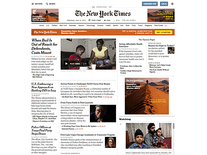This is a blurry, small, square-proportioned screenshot from the New York Times online website. The image is hazy but discernible by the visible "New York Times" title at the top. The webpage is adorned with a couple of advertisements along the top, and below these ads are clickable section headers. The layout is divided into four columns containing five images, where one image appears to be part of the advertisement at the top, alongside several snippets of articles. There are at least eight partial articles displayed, and potentially up to four additional links that may lead to other articles.

In the main image, the scene depicts a domestic indoor setting featuring a mother and child seated at a coffee table. Lower on the page, another article has an image showing a high-contrast profile of a person, illustrating dramatic lighting. Another photograph features a family scene with a man and two children indoors, possibly on a couch; one child is sitting on his lap. The final discernible photo is a headshot of an individual illuminated with dramatic lighting.